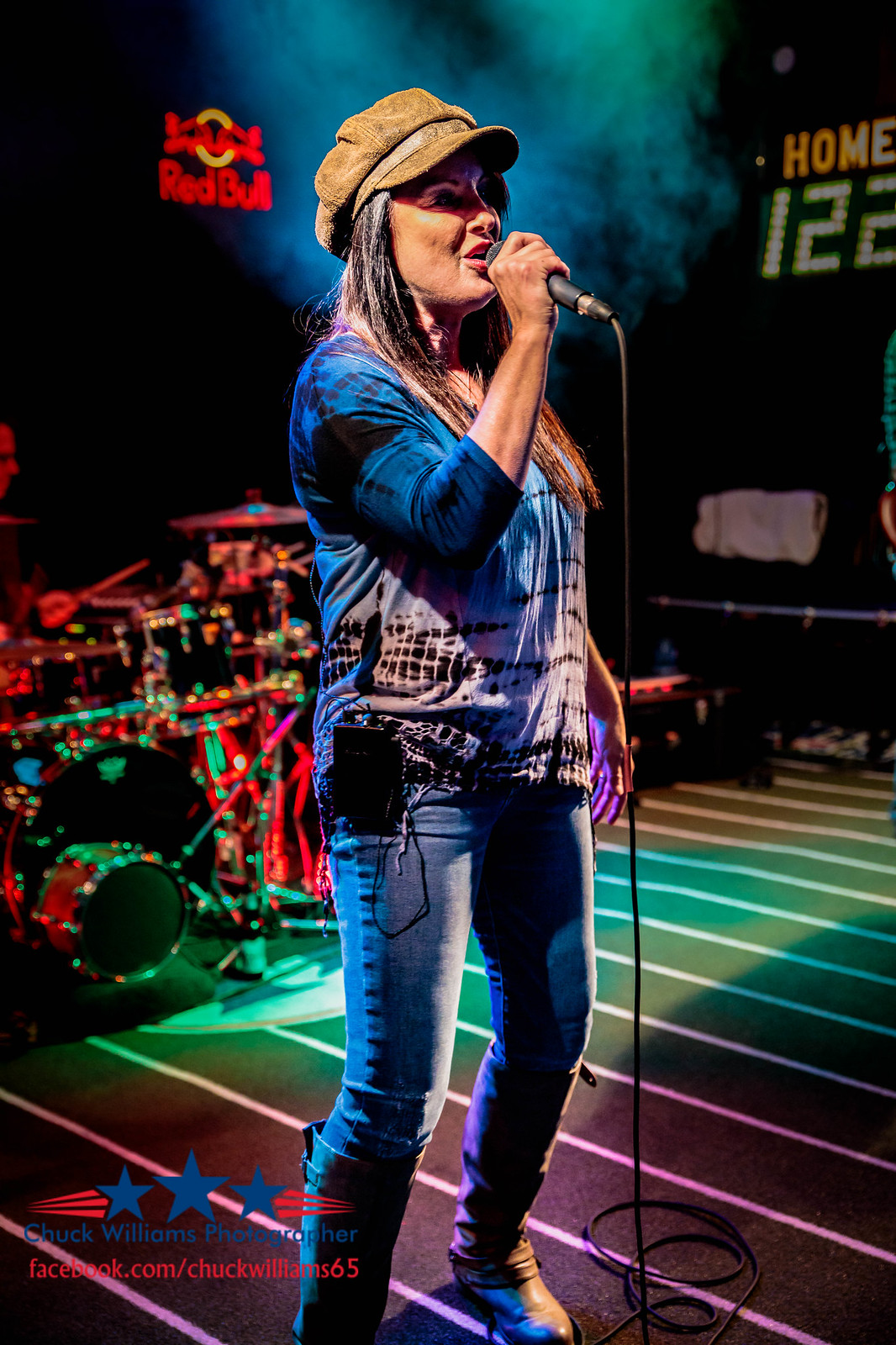In this detailed image, we observe a woman standing center stage in a dimly lit indoor venue, likely a bar or club, with a soft or carpeted surface underfoot. This setting is accentuated by black and white striped patterns across the stage, giving it a sports motif theme. The woman, with long straight brown hair featuring shades of blonde and almost white highlights, dons blue jeans, a blue and white tie-dye blouse, a light brown brimmed hat, and sneakers. She is captured singing into a microphone, holding the audience's attention.

Directly behind her, slightly to the left, is a man playing a drum set. The background features a black wall adorned with signage, including a prominent illuminated Red Bull logo. To the right of the woman, viewers can see a scoreboard prominently displaying a home score of 122 in white numbers, further enhancing the sporty ambiance. The colors in the scene span black, red, yellow, green, brown, blue, gold, and silver, contributing to the vibrant yet moody atmosphere. In the bottom left corner, a watermark reads "Chuck Williams photographer" in blue text accompanied by three blue stars, marking the image's provenance.